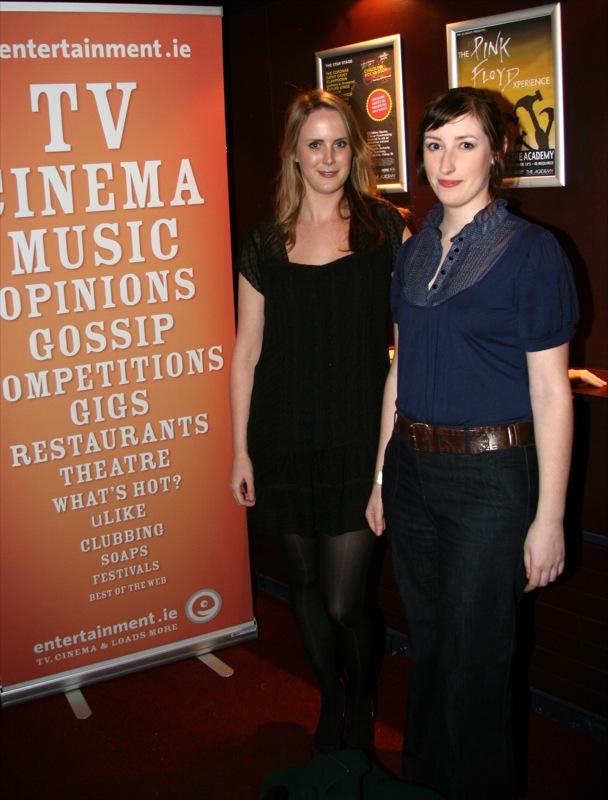The image features two women standing next to each other in the center, both smiling and looking at the camera. The woman on the left is wearing a black cocktail dress and has blondish-reddish hair. To her right, the woman is dressed in black pants with a brown leather belt and a blue short-sleeved button-down blouse; she has short brown hair. They are positioned in front of a prominent orange sign with white text that reads: "Entertainment.ie TV, Cinema, Music, Opinions, Gossip, Competitions, Gigs, Restaurants, Theater, What's Hot, You Like, Clubbing, Soaps, Festivals, Best of the Web." The setting appears to be indoors, possibly at a movie theater or entertainment venue, with a red carpeted floor and a red wall in the background. The atmosphere is vibrant, highlighted by the mixture of colors including orange, white, red, blue, black, and tan.